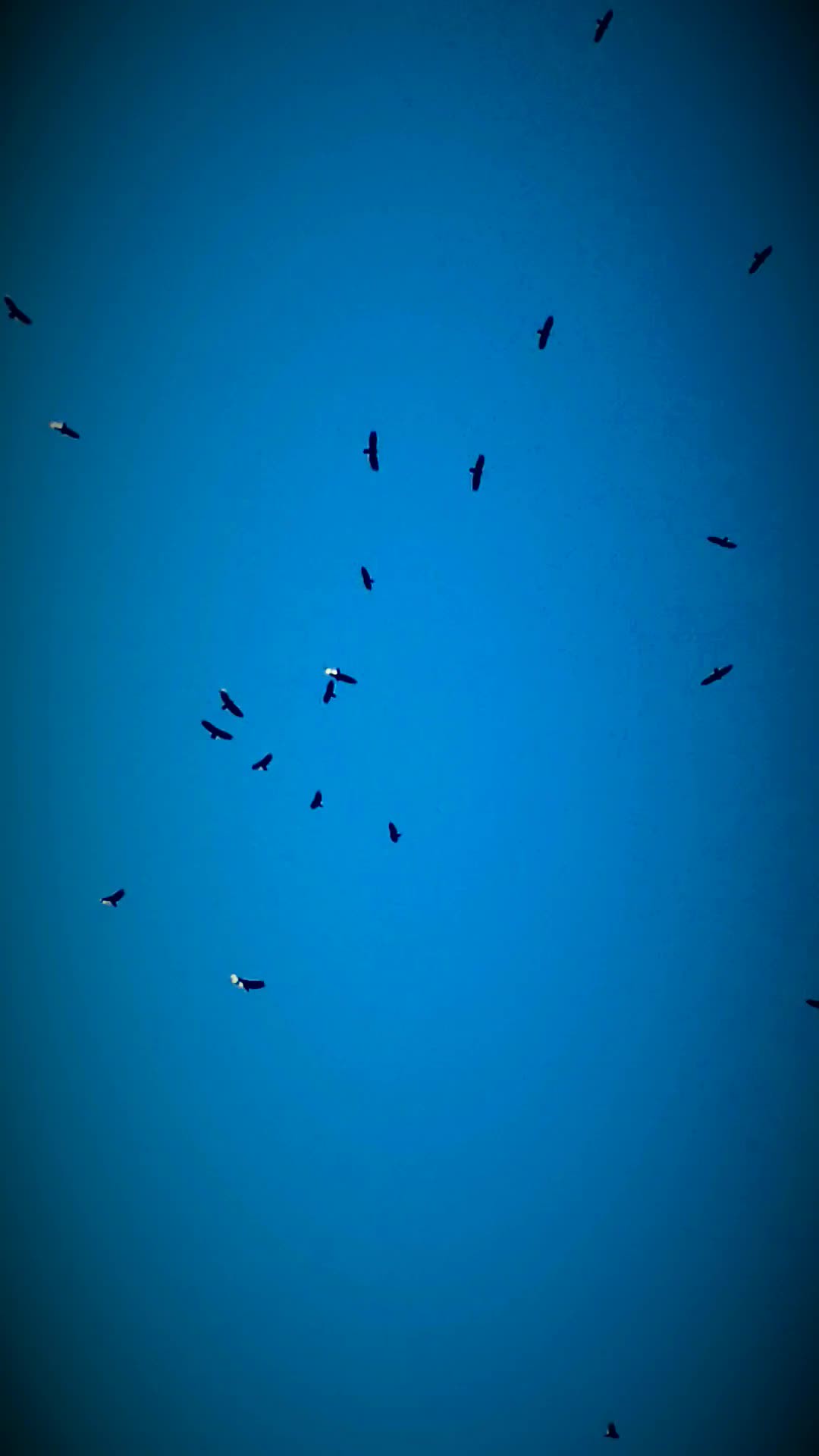A vertical photograph, likely taken with a phone, captures a striking view of a clear blue sky from the ground perspective. The image's long aspect ratio and an applied filter create a dramatic effect, darkening the four corners and fading towards the center, drawing the viewer's attention to the cluster of silhouetted birds. Approximately 15 to 20 birds, perhaps hawks or crows, are scattered and circling in the sky. Their outstretched black wings and occasional white markings are discernible, though the birds remain too distant for precise identification. The deep blue sky, accentuated by the vignette effect and devoid of any clouds, provides a stark, serene backdrop to the dynamic scene of the birds in flight.